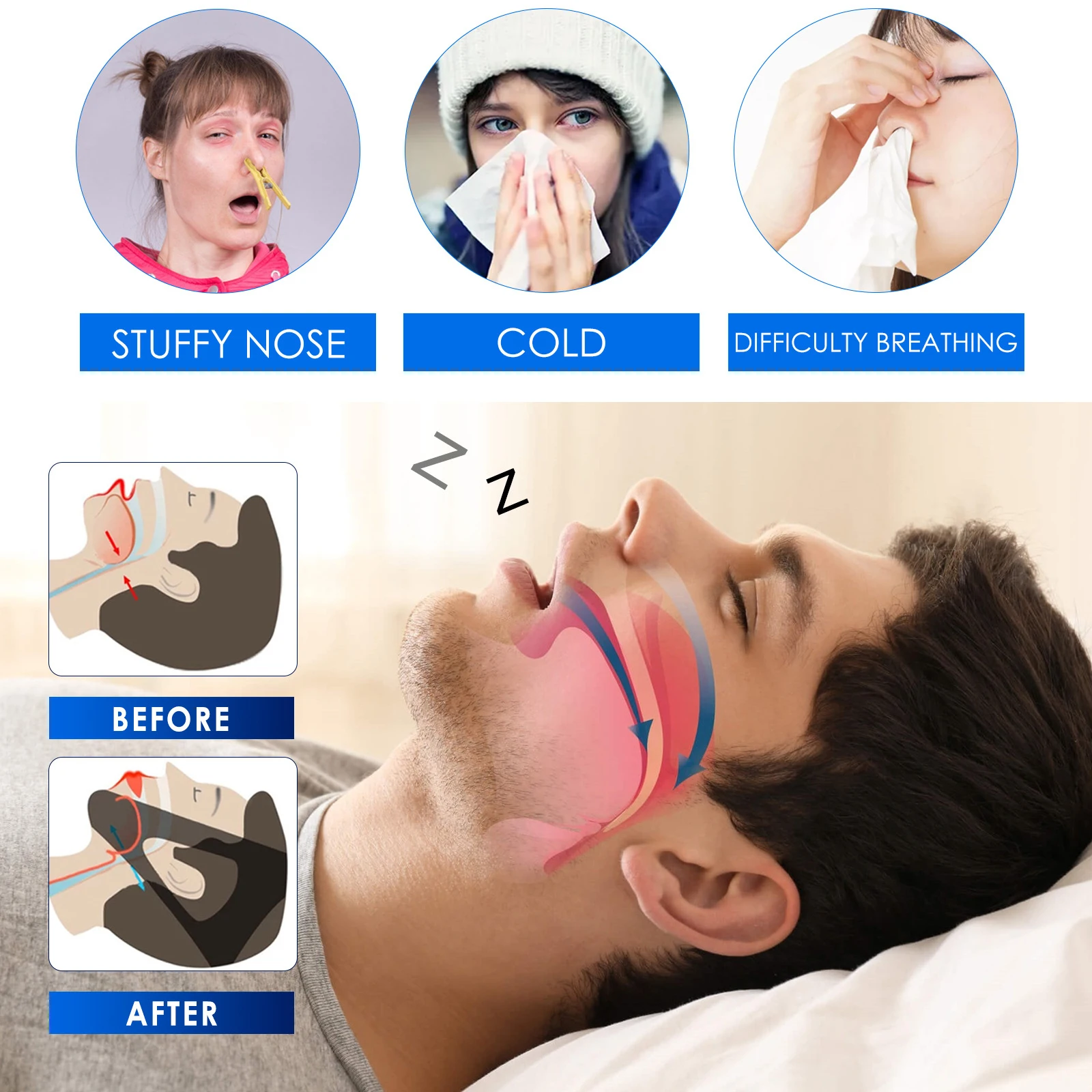The image serves as an advertisement focused on addressing breathing issues, particularly in the context of a cold or nasal congestion. At the top of the image, three circular pictures depict different symptoms. The first circle shows a woman with a clothespin on her nose, labeled "stuffy nose" in white text against a blue background. The second circle features a woman blowing her nose, labeled "cold." The third circle displays a distressed woman with tissues stuffed up her nostrils, holding her sinuses, and labeled "difficulty breathing."

Below these circles, a man with black hair is seen lying on a white pillow. His eyes are closed, and Z's are emanating from his mouth, indicating snoring. Pink, red, and blue arrows illustrate the airflow from his nose and mouth to his throat. Next to this image, two smaller pictures labeled "before" and "after" demonstrate the effectiveness of the advertised solution. The "before" image shows the man with his mouth open, experiencing difficulty breathing. The "after" image showcases a brown gadget that holds his mouth closed, facilitating improved nasal breathing and reducing snoring.